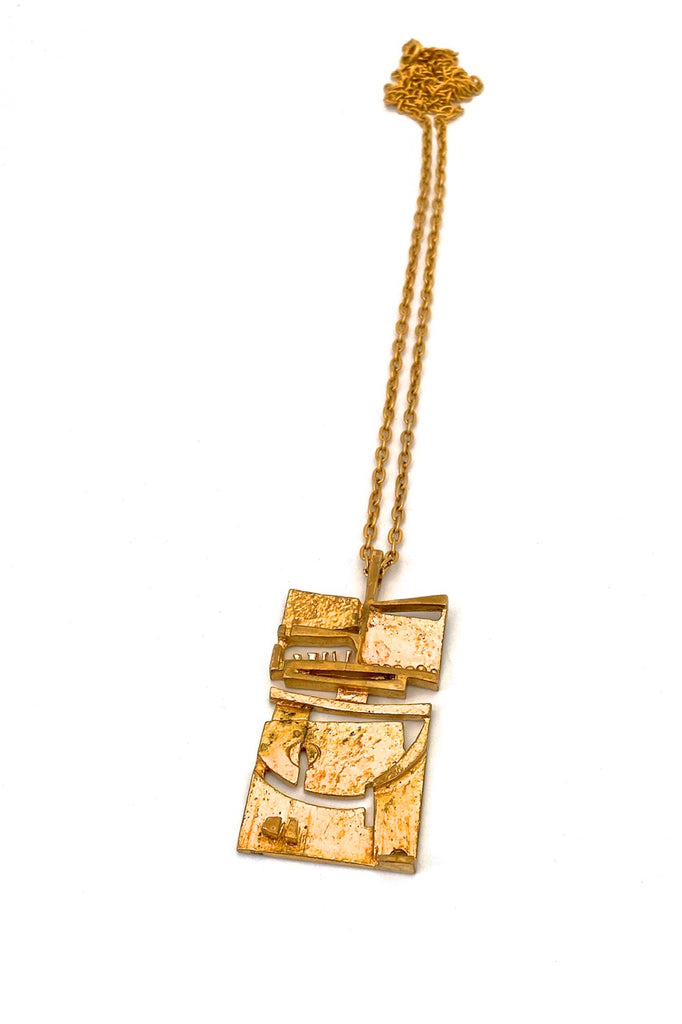The image features a distinctive golden necklace, likely made from a heavy gold-colored chain that gathers at the top before splitting into two straight lines. The pendant or charm hanging from the chain is a complex amalgamation of irregular and interconnected pieces, contributing to a rectangular but fragmented overall shape. This pendant has several openings and gaps scattered throughout, with some appearing almost smile-like or toothed. The top of the pendant curves slightly downward while the bottom remains flat and even. The entire composition looks ancient and artisanal, reminiscent of an artifact, presented against a clean, white background.